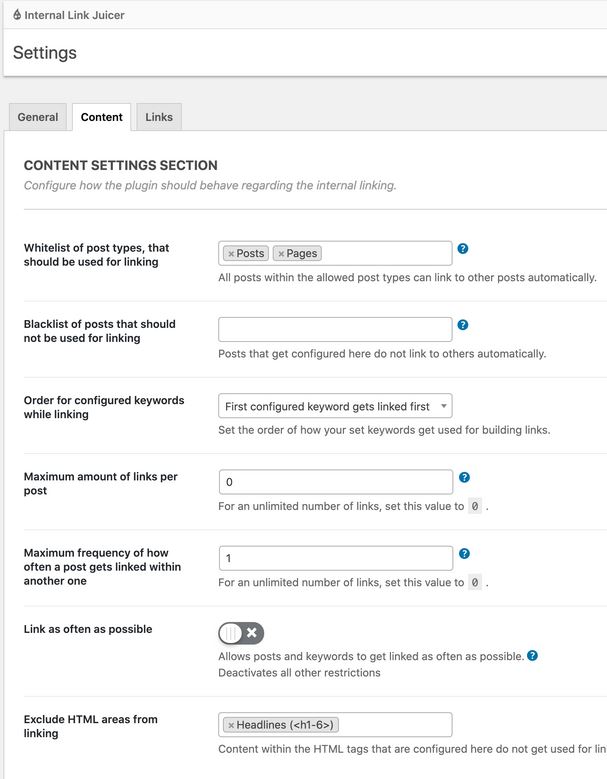The website image displays a user interface for configuring an "Internal Link Juicer" plugin. The central graphic is a teardrop-shaped icon. The settings panel is predominantly black and is divided into various sections, with "Content" being highlighted. The interface shown is a web browser window featuring the "Content Settings" section where users can configure how the plugin handles internal linking.

Key configurations within this section include:

1. **Whitelist of Post Types**:
   - **Label**: "Whitelist of post types that should be used for linking."
   - **Current Setting**: "Posts and Pages" are listed in a white box.
   - **Function**: Allows all posts within these post types to automatically link to other posts.

2. **Blacklist of Posts**:
   - **Label**: "Blacklist of posts that should not be used for linking."
   - **Current Setting**: A white box for entering specific posts.
   - **Function**: Posts configured here do not automatically link to others.

3. **Order for Configured Keywords While Linking**:
   - **Label**: "First configured keywords get linked first."
   - **Description**: Users can set the order of keywords to be used for building links.

4. **Maximum Amount of Links per Post**:
   - **Current Setting**: Set to "0" (indicating unlimited links).
   - **Function**: Users can change this value to limit the number of links per post.

5. **Maximum Frequency of Post Linking**:
   - **Current Setting**: Set to "1".
   - **Function**: Determines how often a post gets linked. For unlimited linking, this value can be set to zero to allow links as frequently as possible.

6. **Slider for Link Frequency**:
   - **Current Status**: Off.
   - **Function**: Allows posts and keywords to be linked as often as possible, deactivating all other restrictions.

7. **Exclude HTML Areas from Linking**:
   - **Label**: "Exclude HTML areas from linking."
   - **Details**: Areas such as headlines and content within specific HTML tags that are configured here will not be used for linking by the LIM (Link Juice Management).

This detailed configuration guide helps users to manage the behavior of their linking strategy effectively, ensuring precision and control over the internal links within their website.